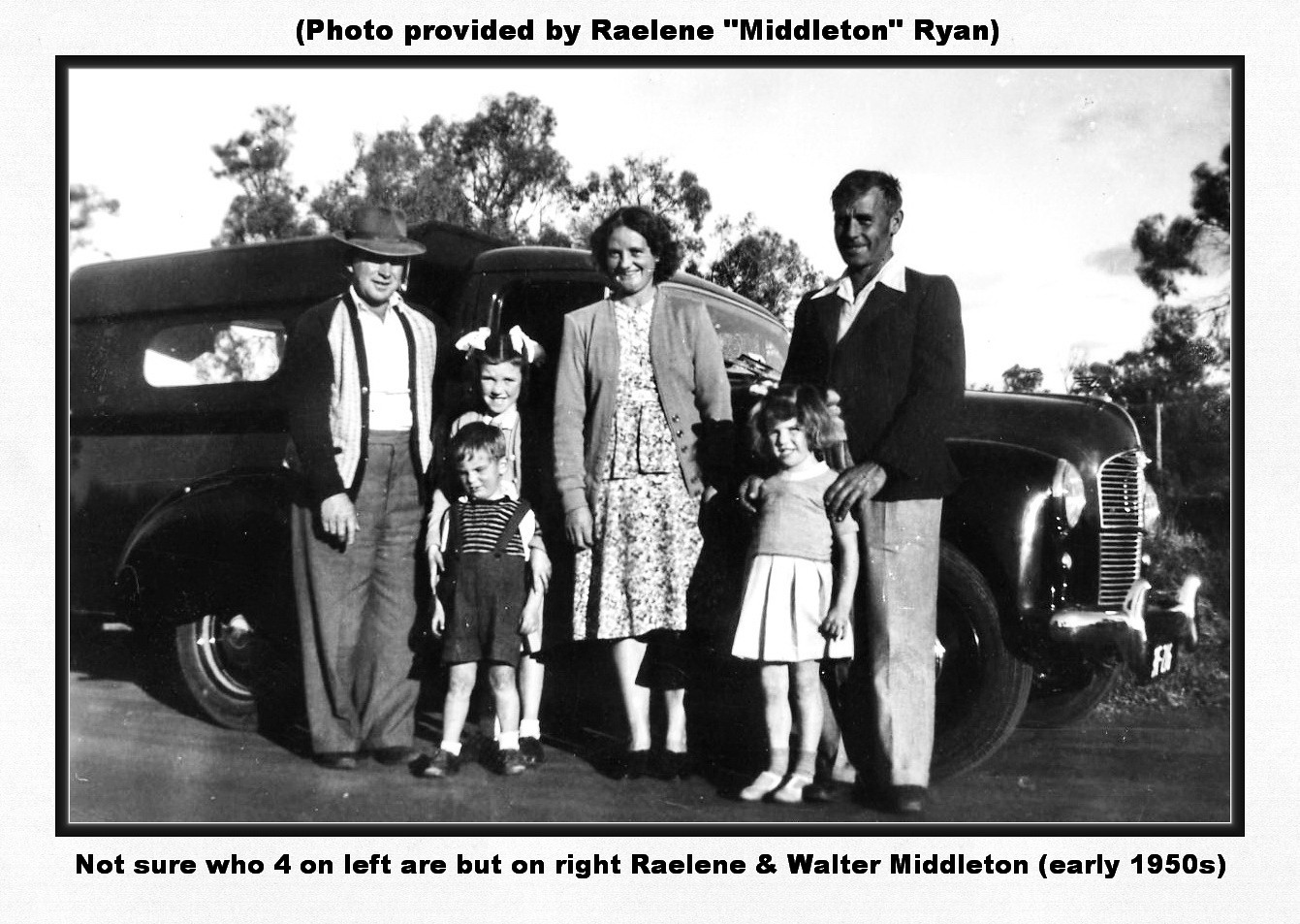The vintage black-and-white photograph, taken in the early 1950s, depicts a family standing in front of a classic, solid black truck characterized by its domed headlights, rounded hood, and fenders, which suggests it dates back to the late 1940s or early 1950s. The family consists of six people: an older man on the far left wearing a fedora, a white and black jacket, gray pants, and a white button-up shirt; he resembles the dad from the Waltons and appears to be in his late 40s. Standing next to him is a woman dressed in a floral dress and jacket. To her right are three children; a little boy in a striped shirt and overalls, and two girls dressed in dresses, one with ribbons in her hair and the other with her hair in ponytails. On the far right is another older man, balding, dressed in a black jacket and a white button-up shirt with a butterfly collar. The background features some trees and an overcast sky. The top of the photograph is labeled, "Photo provided by Raylene Middleton Ryan," and the bottom caption reads, "Not sure who the four on the left are, but on the right, Raylene and Walter Middleton, early 1950s."